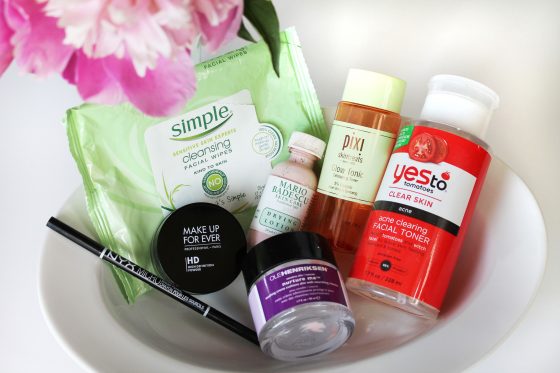**Detailed Caption:**

An indoor, color close-up photograph captures the contents of a white ceramic bowl filled with various skincare and beauty care items. The bowl contains about seven to eight products, arranged meticulously. Starting from the top left and moving right:

1. **Top Left Corner**: A green rectangular flat pack labeled *"Simple"* with green text below reading *"Cleansing Facial Wipes"*.
2. **Slightly Diagonally to the Right**: A small bottle with pink liquid, capped with a clear top. The white label reads *"Mario Badescu"* and mentions *"Lotion"* in smaller text below.
3. **Directly Right**: A slightly larger clear bottle with a yellow cap and label, inscribed in gold lettering *"Pixi"*.
4. **Further Right**: The largest container, a cylindrical clear plastic bottle with a red label featuring a white rectangular center. The text in the white rectangle reads *"Yes To"* in black and *"Clear Skin"* in smaller font below.
5. **Foreground, Center**: A small glass bottle, around an ounce and a half in size, with a purple label that is too blurred to decipher.
6. **Left Center, Facing Camera**: A small circular container labeled *"Make Up For Ever"*.
7. **Diagonal Bottom Left Edge**: A black eyeliner extending out of the bowl towards the left edge.

Additionally, a pink flower with half of its bloom visible, light pink center, and darker pink petals graces the upper left corner of the image, adding a touch of elegance to the scene.